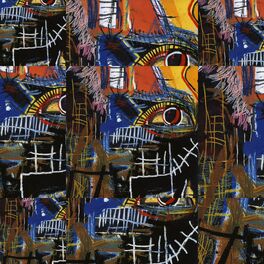This digital artwork is a complex and intense abstract painting characterized by its chaotic composition and vibrant colors. The central motif appears as a window-like structure surrounded by a repeated pattern of the same image, which has been tiled incorrectly in a grid of about 12 imperfect squares. The background is primarily black, adorned with white lines and various patterns that contribute to its busy and somewhat off-kilter appearance.

Prominent colors include reds, yellows, blues, browns, and blacks, with some elements resembling reeds or fences amidst the clashing hues. Two bands of patterned imagery run vertically through the left and right center of the piece, featuring slightly dark backgrounds. Yellow structures comprising multiple squares and lines dominate these areas, overlaid with pink waves.

One particularly striking feature is an eyeball situated between these patterned bands, showcasing yellow whites, a white and red iris, a black pupil, and black eyelashes against a yellow backdrop. Below this, there are sets of white numeral markings, Japanese gate structures, and a sequence of white lines arranged like railroad tracks curving upward and to the right. Splotches of blue accentuate the left side of these structures.

Overall, the painting's myriad of lines, splotches, and geometric forms give it a surreal and chaotic appearance, blending dark tones with bursts of bright color.